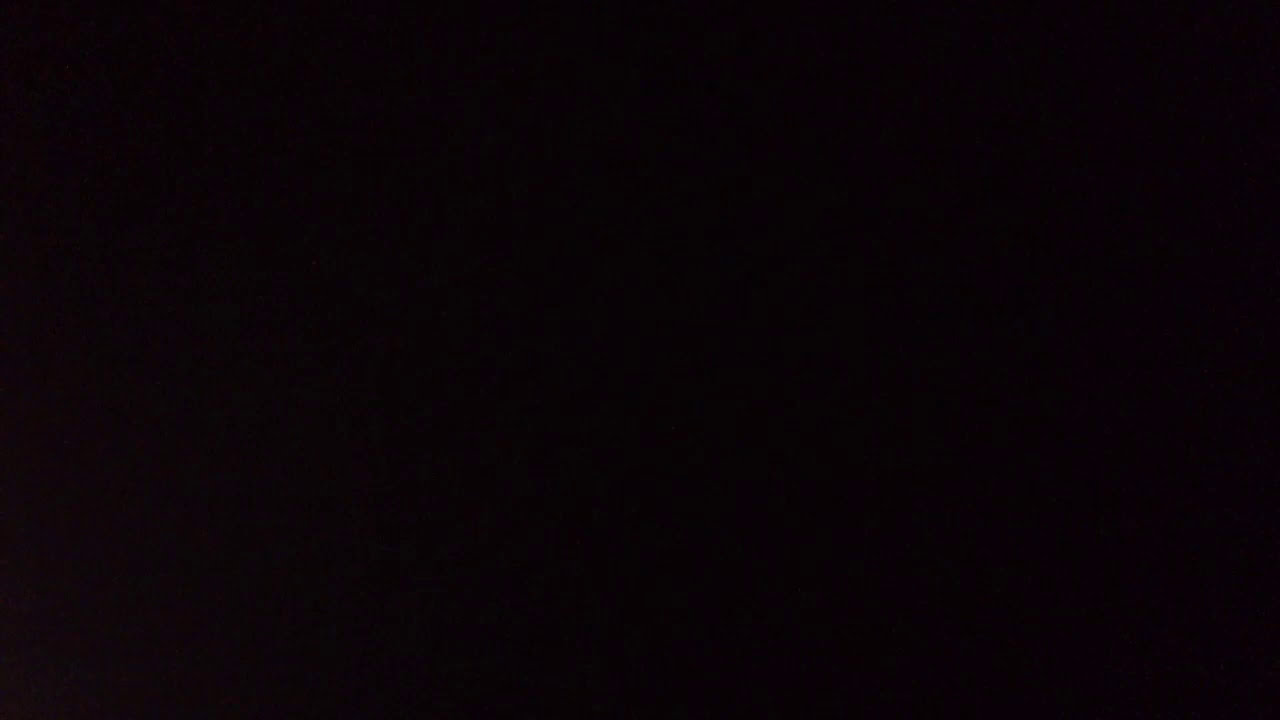This image depicts a completely black rectangle with no discernible shapes, text, or frames. The entirety of the image is uniformly dark, covering every inch with a solid black color. Upon closer inspection, there appears to be a subtle static throughout the image, predominantly green, scattered sporadically across the frame. This static might be an artifact from the monitor display or inherent to the image itself. Overall, the image presents as a pure, unbroken black rectangle, suggesting it could be a screenshot taken just before or after a video or potentially a photo with an inactive camera lens.